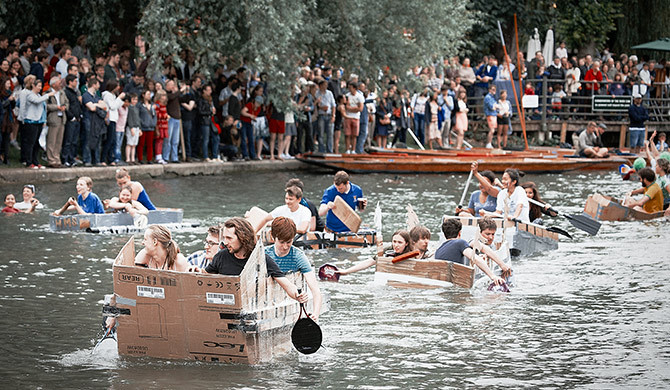The image captures a lively outdoor event during the daytime, where participants are engaging in a spirited cardboard boat race on a dark grey lake. The contestants, dressed in summer attire, are seen laughing and having fun as they paddle their handmade cardboard boats, some using unconventional tools such as tennis rackets, flat pans, or their hands. The boats, primarily brown, display various sizes, often resembling large cut-up boxes. A lush, leafy branch dripping into the scene at the top middle of the image adds a sense of nature to the vibrant activity.

In the background, a sizable crowd of spectators stands along the edge of the water, cheering, taking photos, and enjoying the spectacle. The observers are densely packed, some shielded by overhanging trees, and extend along a concrete bank and dock railing of what appears to be a river. The setting, bathed in natural light, suggests it may be a pleasantly warm day, albeit with a slight chance of rain or breeze, as indicated by a few individuals donning light jackets. Overall, the photograph exudes a sense of community, recreational sport, and playful creativity against a backdrop of enthusiastic support.